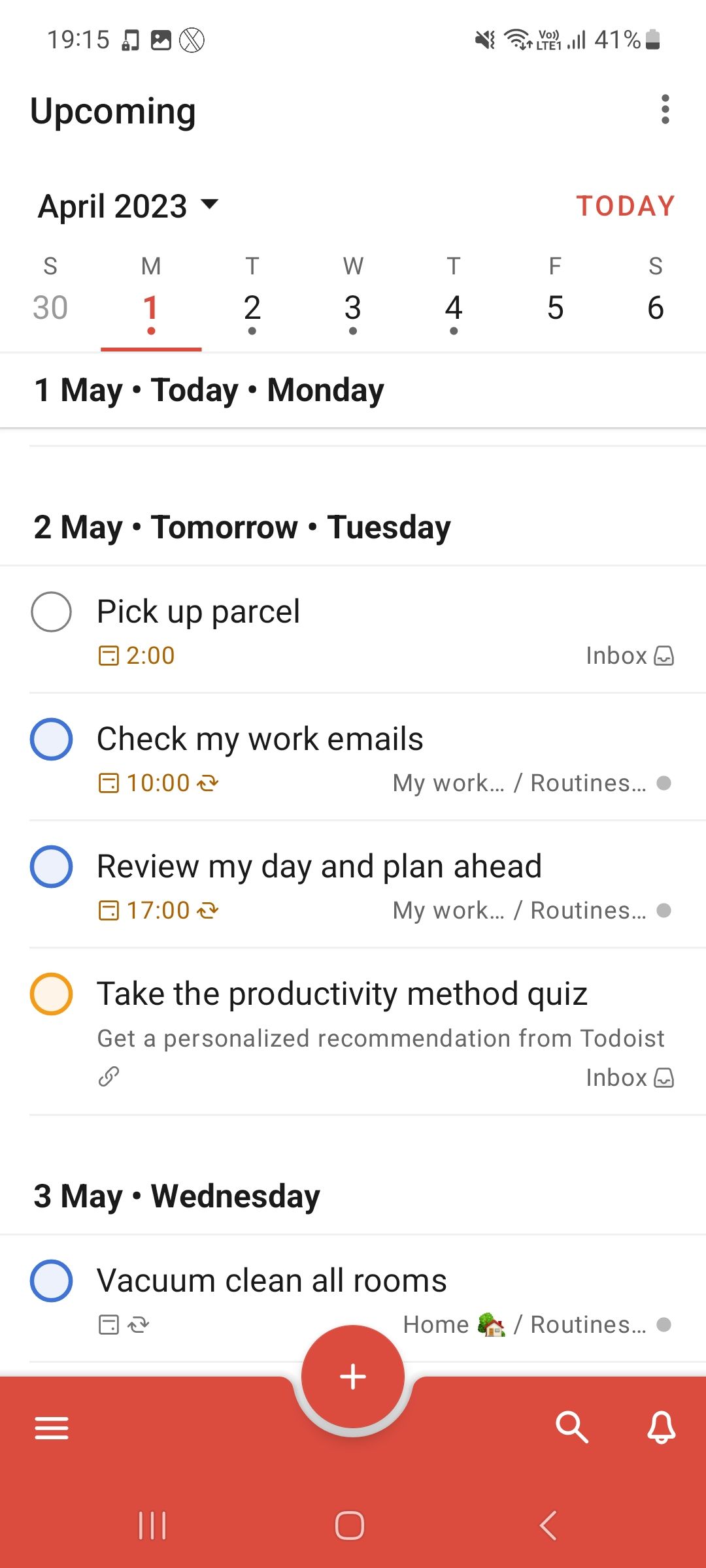A screenshot of a computer screen showing a detailed agenda and calendar. At the top, there's a header labeled "Upcoming." The current time displayed is 19:15, and icons are present in both the upper left and upper right corners. Below the header, it indicates the month as "April 2023" and lists the days of the week with corresponding dates: Sunday (30), Monday (1), Tuesday (2), Wednesday (3), Thursday (4), Friday (5), and Saturday (6).

Highlighted prominently, it says "1 May today Monday" and "2 May tomorrow Tuesday." Further down, action items for May 1st are listed: "Pick up parcel," "Check my work emails," and "Review my day and plan ahead." The final task for May 2nd is "Take the productivity method quiz." At the very bottom, "3 May Wednesday" is displayed, indicating the date progression.